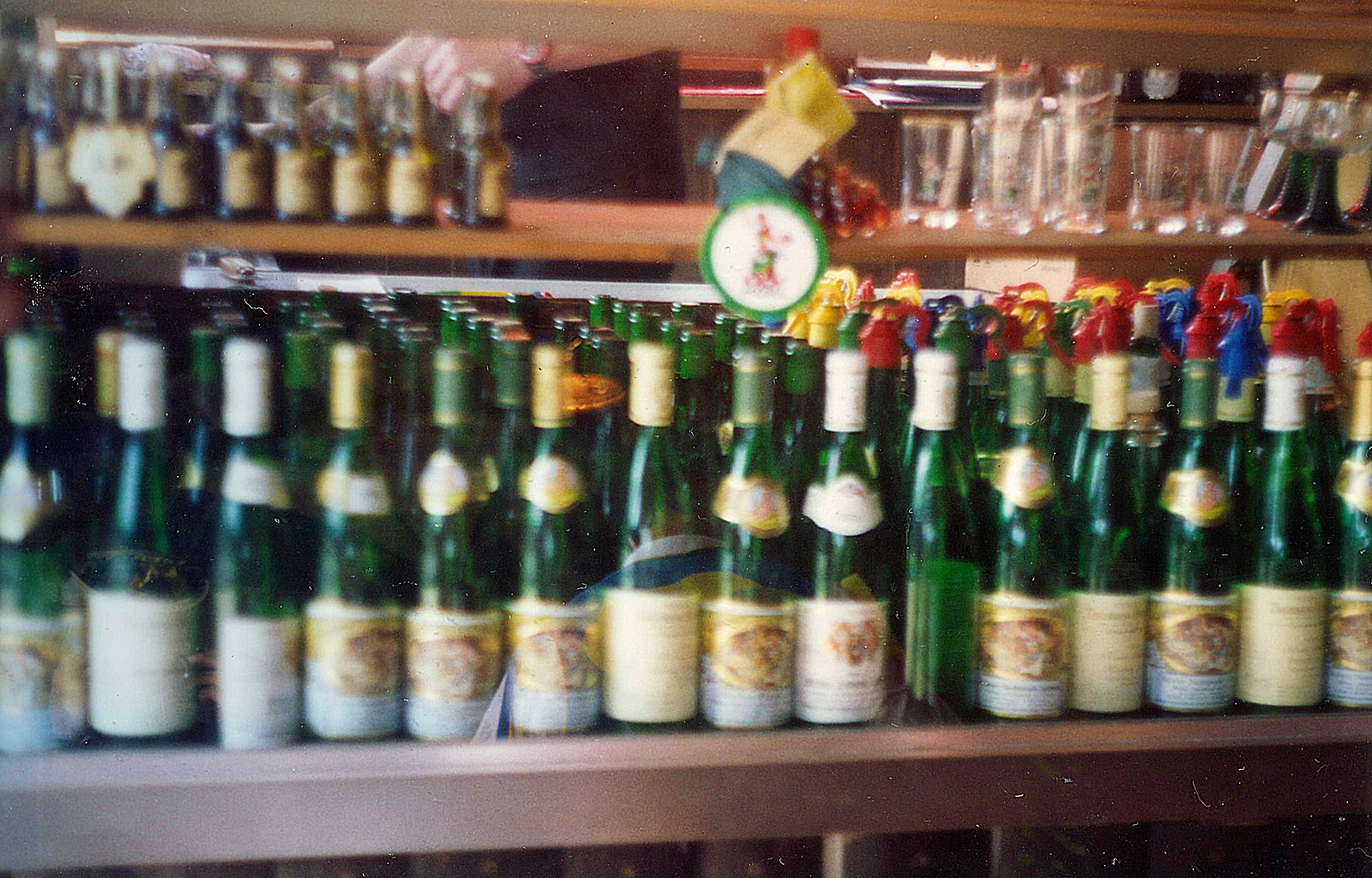This photograph, though blurry, captures the interior of a bar featuring an organized display of numerous bottles on two shelves. The primary focus is on the bottom shelf, which is densely packed with green beer bottles. Each bottle sports similar beige and gold labels around its bottom half, with some also featuring thinner gold labels near the neck. The bottle caps vary in color, including white, green, and gold, and the right half of this bottom shelf showcases bottles with colorful stoppers—red, blue, yellow, and green. Above, the upper shelf exhibits a variety of items: the left side holds miniature or brown bottles with beige labels, while the right side is arrayed with shot glasses. The shelves themselves transition in color from grey on the left to light and dark brown on the right, lending a rustic wooden ambiance to the scene. Additional colors in the background, such as red and blue, hint at more bar essentials and decor, further accentuating the eclectic yet systematic nature of this bar setup.